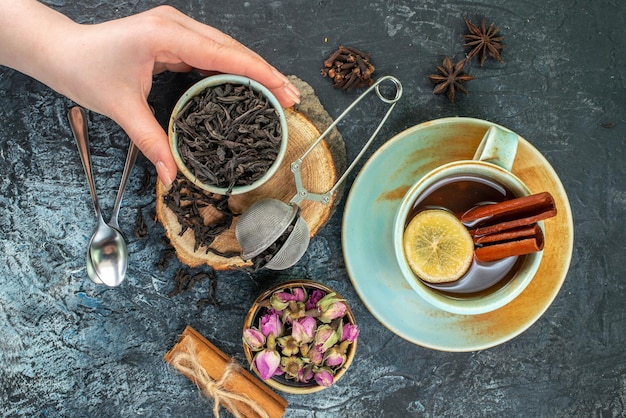A top-down view captures an elaborate breakfast tea ceremony set against a textured dark gray background. Central to the composition is a small ceramic cup of freshly brewed black tea resting on a slice of a tree stump, held delicately by a hand entering from the upper left. The cup is beautifully decorated with a breakfast flower ceremony motif, floating with a slice of lime or lemon and tubular pieces of cinnamon, exuding an aura of authenticity and floral elegance.

Surrounding the centerpiece are various intricate elements, including two small teaspoons, with one holding a pellet, and a tea strainer placed thoughtfully to the side. A small container filled with dried purple and white flower buds rests in the lower left, adding a touch of natural beauty. Adjacent to this is a scroll, possibly a napkin wrapped in twine, enhancing the rustic charm.

In the upper right corner, two star-shaped pine cones and brown pellets, along with a unique double scoop tool resembling a safety pin, contribute to the detailed arrangement. Beneath the hand, a white ceramic bowl with black herbal elements, possibly tea leaves or spices, sits over a slightly larger brown bowl, intensifying the layered textures. The lower right features a blue and brown plate that holds a teacup with visual accents of floral motifs, concluding this visually rich and meticulously detailed scene.